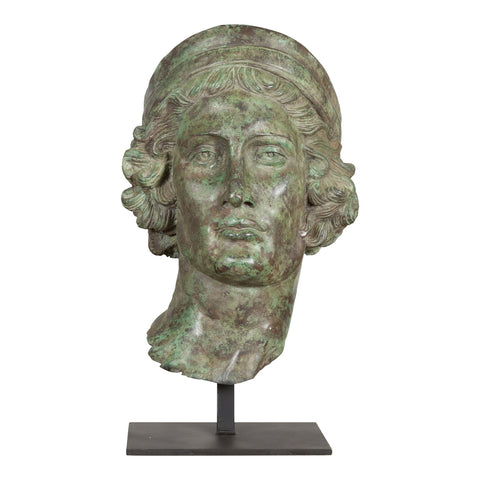The image depicts a highly detailed sculpture, likely found in a museum, featuring the head and neck of a young man. The sculpture is mounted on a sleek, black rectangular stand with a supporting pole in the middle. Rendered in a polished stone resembling marble, its surface showcases an intriguing blend of light brown and jade green hues with possible black inclusions. The man in the sculpture has a rectangular-shaped face with a neutral expression and a long nose. His short, curly hair, which extends to about mouth level, features intricate detailing, further accentuated by what appears to be a headband or a rounded, dome-like hat. The man gazes directly ahead, adding a compelling presence to the piece.